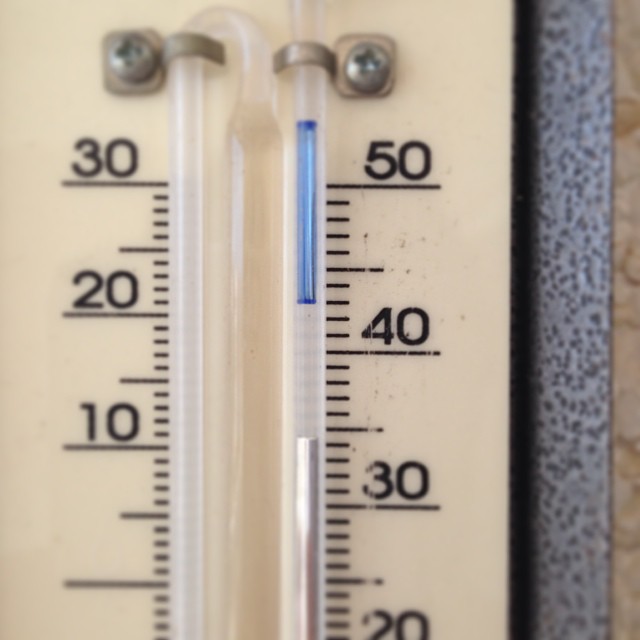The image depicts a rudimentary setup featuring a backdrop of what appears to be plywood. In the foreground, a piece of metal supports a thermometer, giving an initial impression of an outdoor setting. The thermometer has two distinct columns. The left column appears to be an empty tube and is secured at the top with Phillips head screws and small silver loops. It bears the numbers 30, 20, and 10 but no other markings, indicating a potentially incomplete or partially functional instrument. The right column, marked with numbers 50, 40, 30, and 20, displays a silver substance reaching up to the 35 mark, above which a blue substance extends from around 44 above the 50 mark, suggesting a possible malfunction or a different type of measurement, such as humidity, rather than temperature. The ambiguity in the instrument's design and markings leaves the precise nature of its measurements unclear.